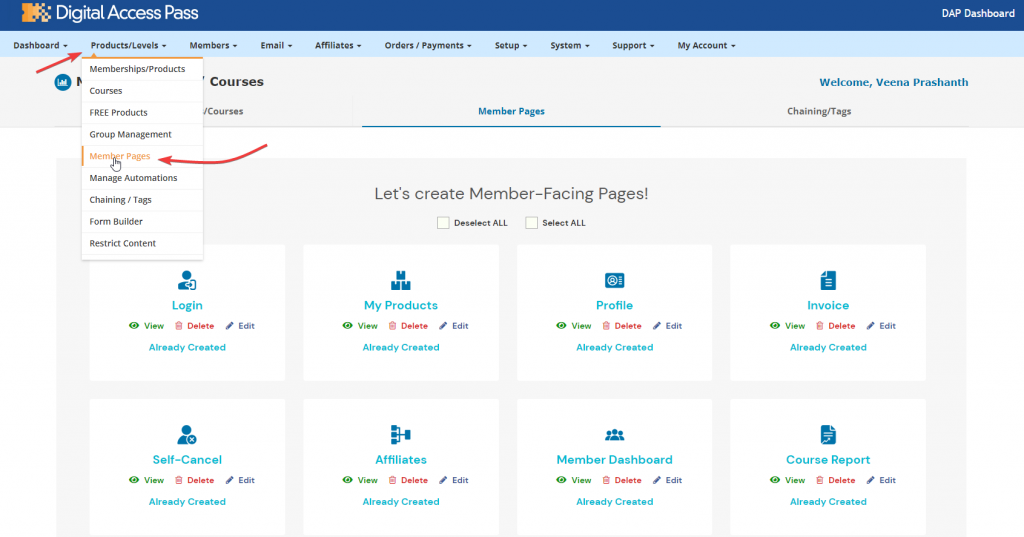The image showcases a computer screen displaying a detailed dashboard of a digital access management system. The interface features a dark blue or navy blue banner at the top, adorned with a distinctive logo: a gold 'M' that gradually disintegrates towards the right. The text "Digital Access Pass" is prominently situated beside the logo, with "DAP Dashboard" appearing on the extreme right.

Directly beneath the banner, a secondary menu highlights various sections including "Dashboard" and "Products/Levels," both of which are drop-down menus. Currently, the "Products/Levels" drop-down menu is expanded to reveal options such as "Memberships," "Products," "Courses," "Free Products," and "Group Management." Additionally, "Member Pages" is selected, displaying further options like "Manage," "Automations," "Chaining," "Tags," "Form Builder," and "Restrict Content."

Below this, a directive reads, "Let's Create Member Facing Pages," indicating the current focus on Member Pages. Eight organizational elements are listed: "Login," "My Products," "Profile," "Invoice," "Self-Council," "Affiliates," "Member Dashboard," and "Course Report." None of these options have been clicked on. 

Options to "Deselect All" or "Select All" are provided for bulk operations. This comprehensive layout allows for versatile management of digital access and member interactions with the platform.